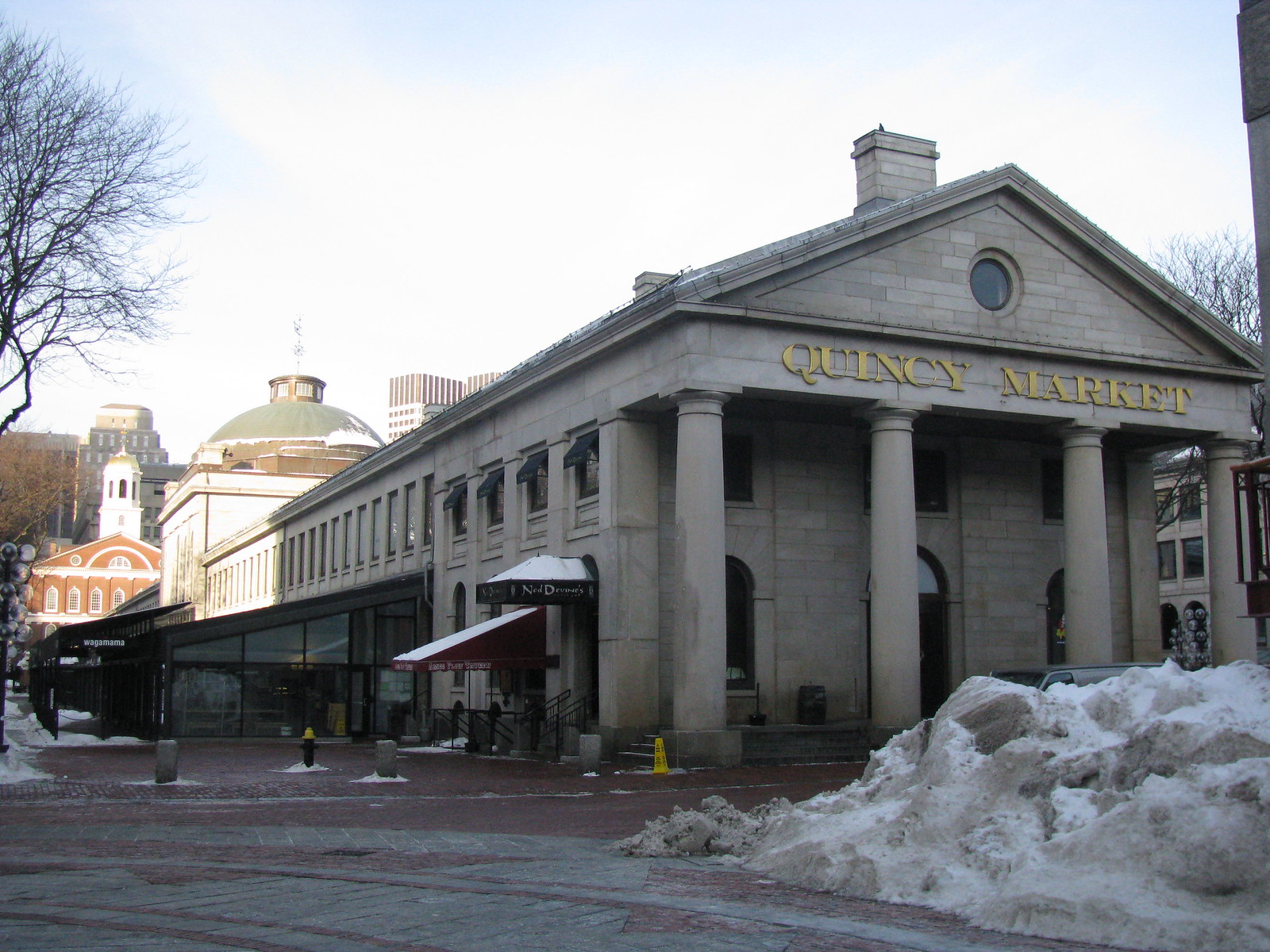The image depicts a large and elegant old building named Quincy Market, prominently located in Boston, Massachusetts. The structure, built from gray stone, features a grand façade with four imposing Roman columns supporting a triangular pediment, giving it a distinctive Greek architectural style. The name "Quincy Market" is emblazoned in gold letters above the entrance. In front of the building, there is a substantial pile of dirty, freshly plowed snow. The photograph also captures a winter setting, evident from the snow and the clear blue sky with scattered white clouds overhead. In the background, you can see traces of historical New England architecture, including a domed building and an old church, adding to the rich historical context of the scene.